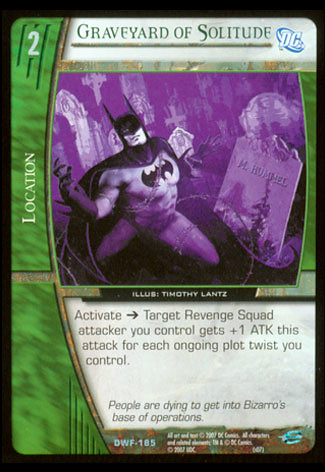The image is of a DC Comics-themed trading card with a distinctive black border surrounding it. On the left side of the card, there's a large green section with the white word "Location." At the top of the card, a white section with green text titles it "Graveyard of Solitude," accompanied by the DC Comics logo in the upper right corner and a white number "2" in the upper left. Below, a purple-tinted image of Batman is depicted in a graveyard, tangled in vines, and surrounded by tombstones. Underneath this illustration, a white section with black text reads: "Activate ⟶ Target Revenge Squad attacker you control gets +1 ATK this attack for each ongoing plot twist you control." The card is Bizarro's base of operations as noted in the flavor text, "People are dying to get into Bizarro’s base of operations."